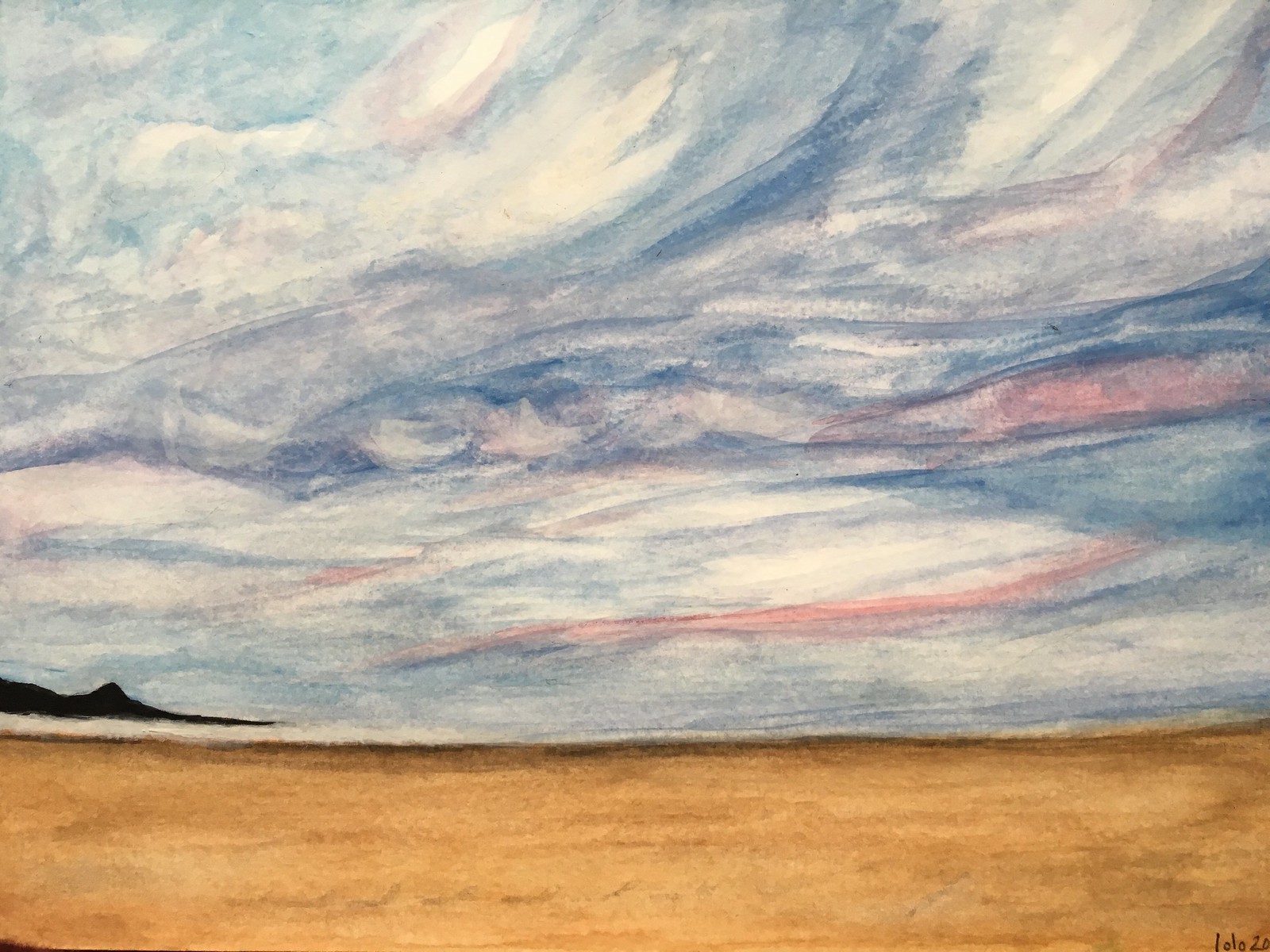This captivating image resembles a painting, depicting a sprawling expanse of brown earth that stretches towards the horizon where a lighter hue emerges. In the distance, a small dark sliver of a hill or mountain punctuates the landscape. The sky above is a dynamic blend of colors, with areas where the white paper beneath the paint peeks through. Various shades of blue dominate the sky, ranging from deep navy to a lighter teal, interspersed with gray clouds, and complemented by streaks of white. Hints of pink grace the sky, concentrated near the middle bottom and faintly extending to the top. Intricately detailed, the scene is both serene and striking. In the bottom right corner, black writing is visible, albeit difficult to decipher. The characters appear to spell "LOLOZO," though the text could potentially include numbers, creating ambiguity in the exact letters or digits shown.